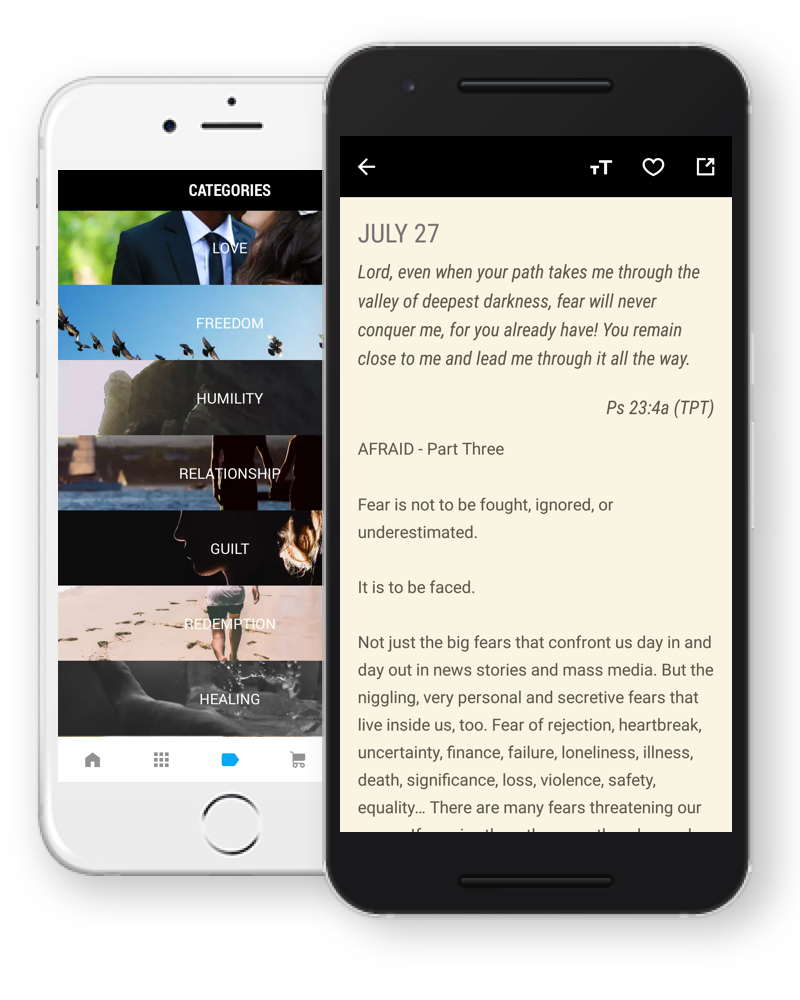The image displays two phone screens showcasing a Bible-themed app. The first screen is from a white phone featuring a circular home button at the bottom. The app's interface reveals a list of categories written in white text on black strips, including "Love," "Freedom," "Humility," "Relationship," "Guilt," "Redemption," and "Healing."

The second screen is from a black phone, highlighting an open section of the app. It shows a devotional reading dated "July 27th," written in dark gray text on a faint yellowish-sandy background. The passage reads: "Lord, even when your path takes me through the valley of deepest darkness, fear will never conquer me for you already have. You remain close to me and lead me through it all the way." This is an adapted version of Psalm 23:4a, with a notation marked "TBD."

Below the scripture, the heading "Afraid - Part 3" introduces a reflective piece on fear. It emphasizes that fear should neither be fought, ignored, nor underestimated, but faced head-on. It mentions various fears that confront us daily—ranging from those highlighted by news stories and media to personal, secret fears like rejection, heartbreak, uncertainty, financial issues, failure, loneliness, illness, death, significant loss, violence, safety, and equality. The text continues but becomes partially obscured, ending with the words "There are many fears threatening our," leaving the rest of the sentence unreadable.